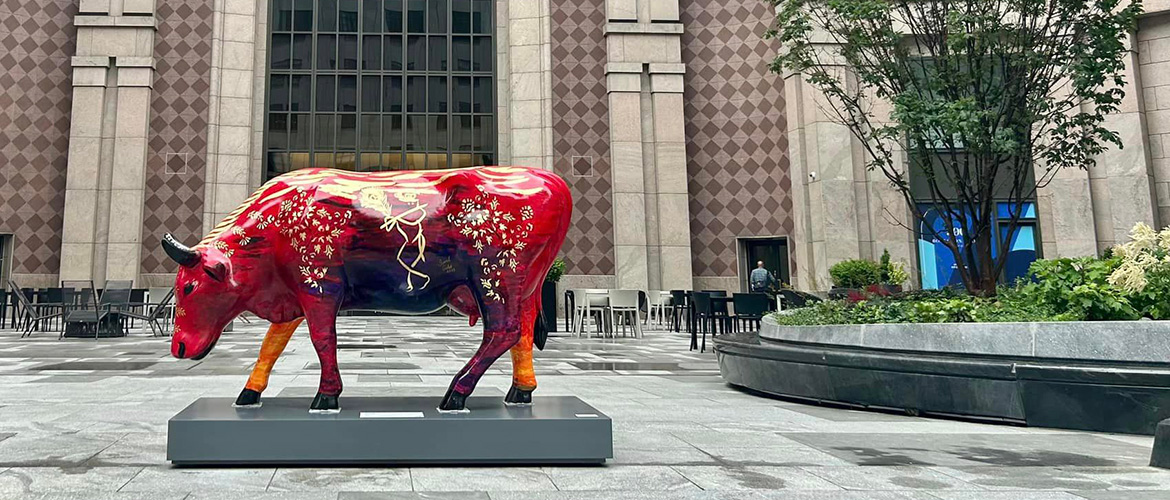This image captures an outdoor plaza in a city area, centered around an ornately decorated red cow statue facing left. The cow, adorned with intricate white patterns and sporting a multi-colored underside and legs, stands on a short gray pedestal bearing labels that likely identify the artwork and the artist. The surrounding area features gray tile flooring.

To the right of the statue, a circular black stone bench encloses a small garden with a tree and other plants, suggesting an outdoor setting. Behind the statue, there is ample seating with tables and metal or mesh chairs, possibly for people to sit, eat, or relax. The backdrop is a large building with a distinctive diamond-shaped tiling pattern, large windows, and columns of marble or stone. This building has multiple doorways, and one doorway appears to have a person entering. The windows reflect the image of the building across the street, adding depth to the urban scene.